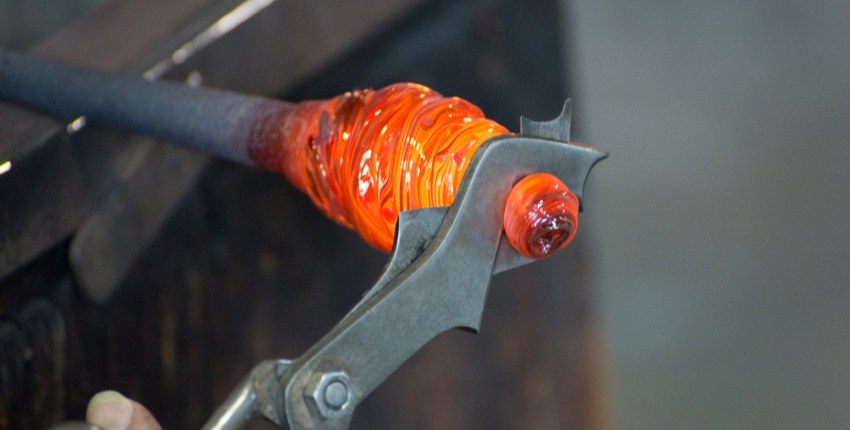In the image, a skilled artisan is meticulously cutting the tip of molten material, which resembles orange-yellowish glass or metal, using metallic shears. The semi-liquid, heated substance is attached to the end of a rod that lies across a metal bar, visible predominantly from the left side. The shears or clamps are gray and the background is deliberately blurred, displaying hues of brown on the left and gray on the right. On the left side, part of a finger or thumb can be glimpsed, hinting at the careful manual dexterity required in this intricate process.